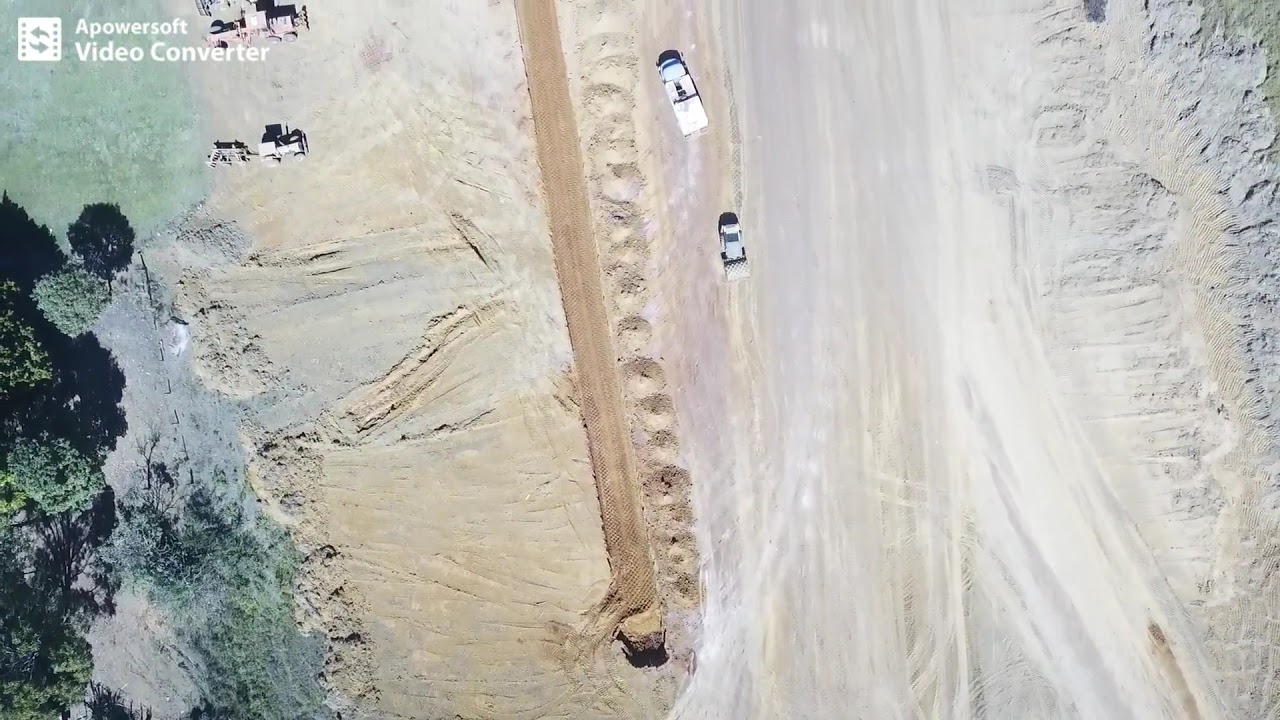An aerial, bird's-eye view of a predominantly sandy landscape, potentially a construction site, occupies the image with its broad expanse of tan and brown hues covering about seven-eighths of the frame. The upper center features two white trucks, while the top left corner shows a couple of tractors amidst this sandy sea. The right-hand section is marked by a more concentrated patch of white sand, possibly indicating rocky terrain. To the far left, a small piece of greenery interrupts the sandy expanse, showcasing some lush green trees and a piece of grass, alongside a dark brown dirt trail running vertically. The only textual element in the image is in the upper right corner, where it reads "A Powersoft Video Converter."